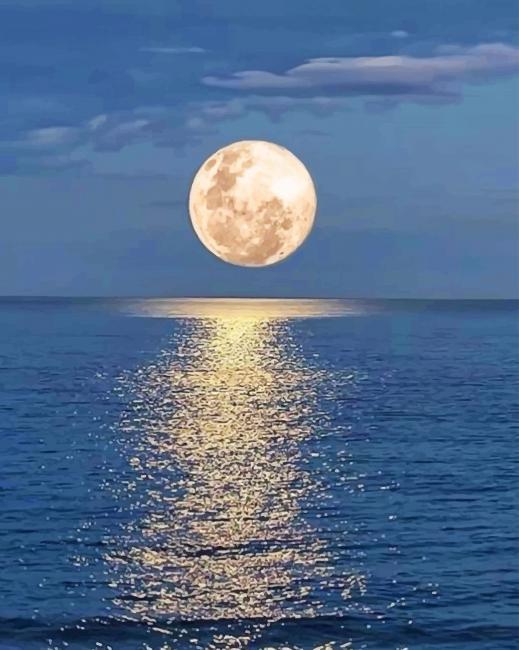Under a deep, mesmerizing blue sky dotted with wisps of white clouds, a gigantic luminescent moon dominates the center of the scene. Positioned almost as if it is gently kissing the horizon, the moon's reflection stretches far and wide across the tranquil ocean below. The water, shimmering in a breathtakingly vivid blue, holds a glistening streak down its center where the moonlight dances and sparkles. Towards the bottom of the image, the water deepens into a darker shade, yet retains its captivating hue. The horizon seems infinite, blending seamlessly with the sky in a boundless expanse of blue, punctuated by the striking, radiant moon embellished with subtle dark spots.